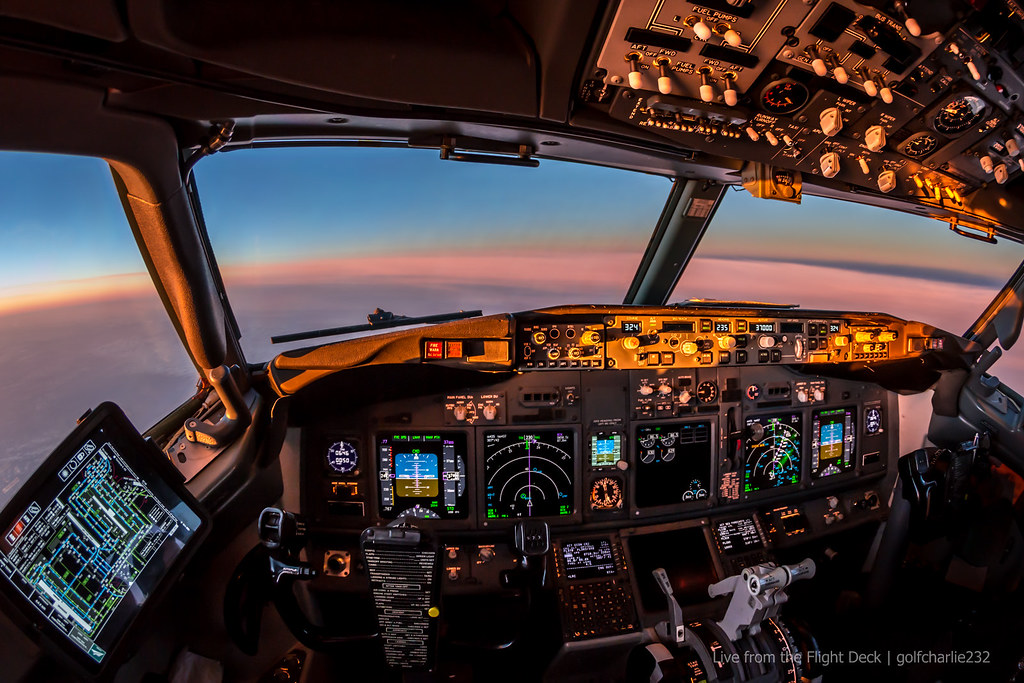The image captures the intricate interior of an airplane cockpit, showcasing the complex array of mechanisms that pilots manage. The cockpit is filled with numerous buttons, switches, dials, and levers, with many controls even situated on the ceiling. Central to the dashboard are five computer screens, including a large one on the left, providing vital flight information. Visible through the four surrounding windows, two at the front and one on each side, is a stunning high-altitude view of a clear blue sky adorned with pinkish, yellow, and beige clouds. The serenity of the sky contrasts with the busy and highly technical cockpit. In the lower right corner of the image, the title "Live from the Flight Deck, Dash Golf Charlie 232" is displayed, emphasizing the live aspect of the scene.